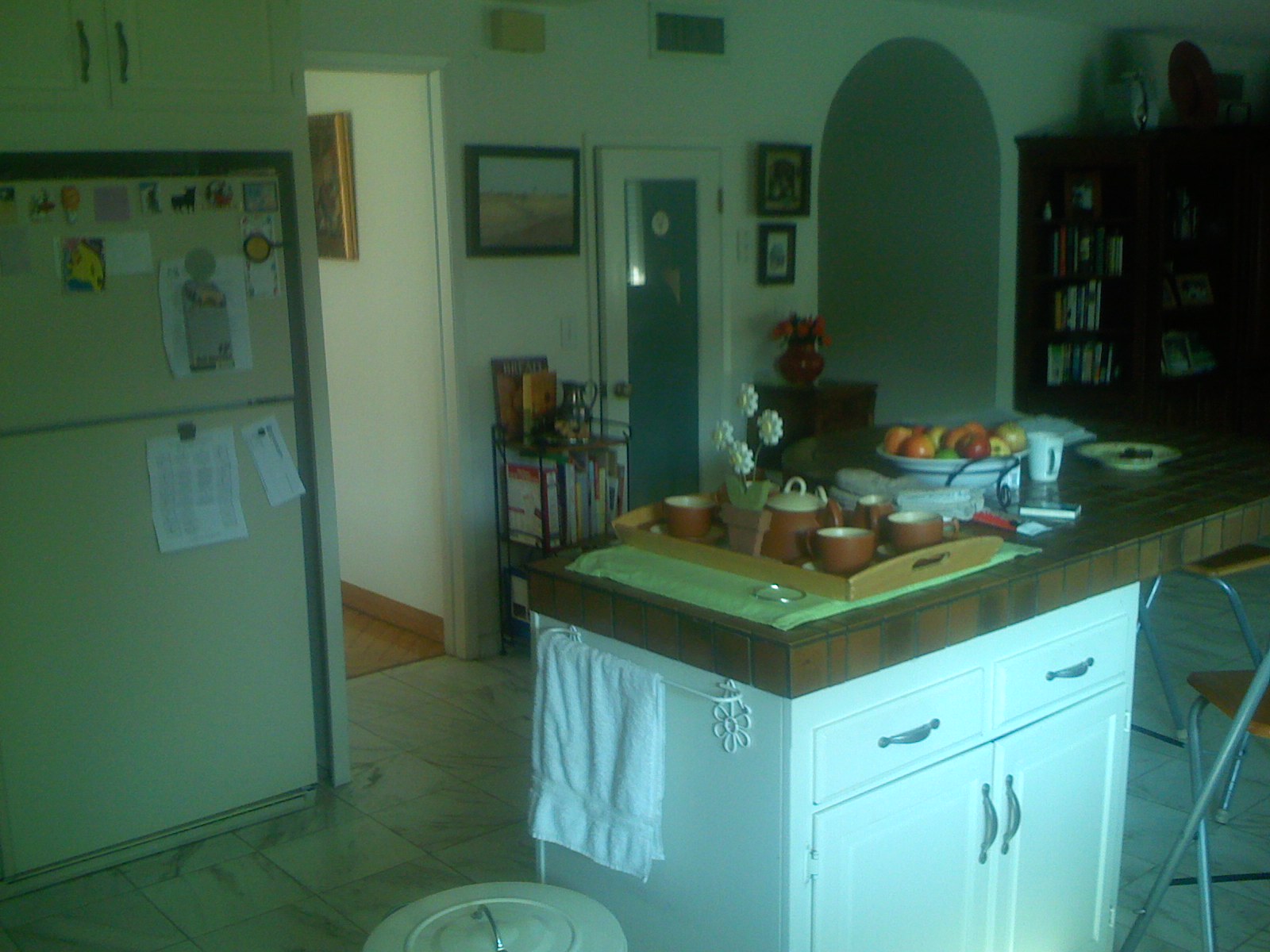Inside the kitchen, an older white refrigerator stands on the left, adorned with several pieces of paper secured by a row of assorted magnets at the top. The refrigerator features a freezer section above and a larger fridge compartment below. Centrally located in the room is an island counter, showcasing a tray that holds several teacups and a plate brimming with a variety of fruits, including apples. Nearby, a set of simple metal foldable chairs are positioned next to the counter. The island also features a few white drawers and supports a small trash can at its bottom left corner, with a white towel neatly hanging from a rack. In the background, bookshelves and a doorway leading to what appears to be the living room are visible.